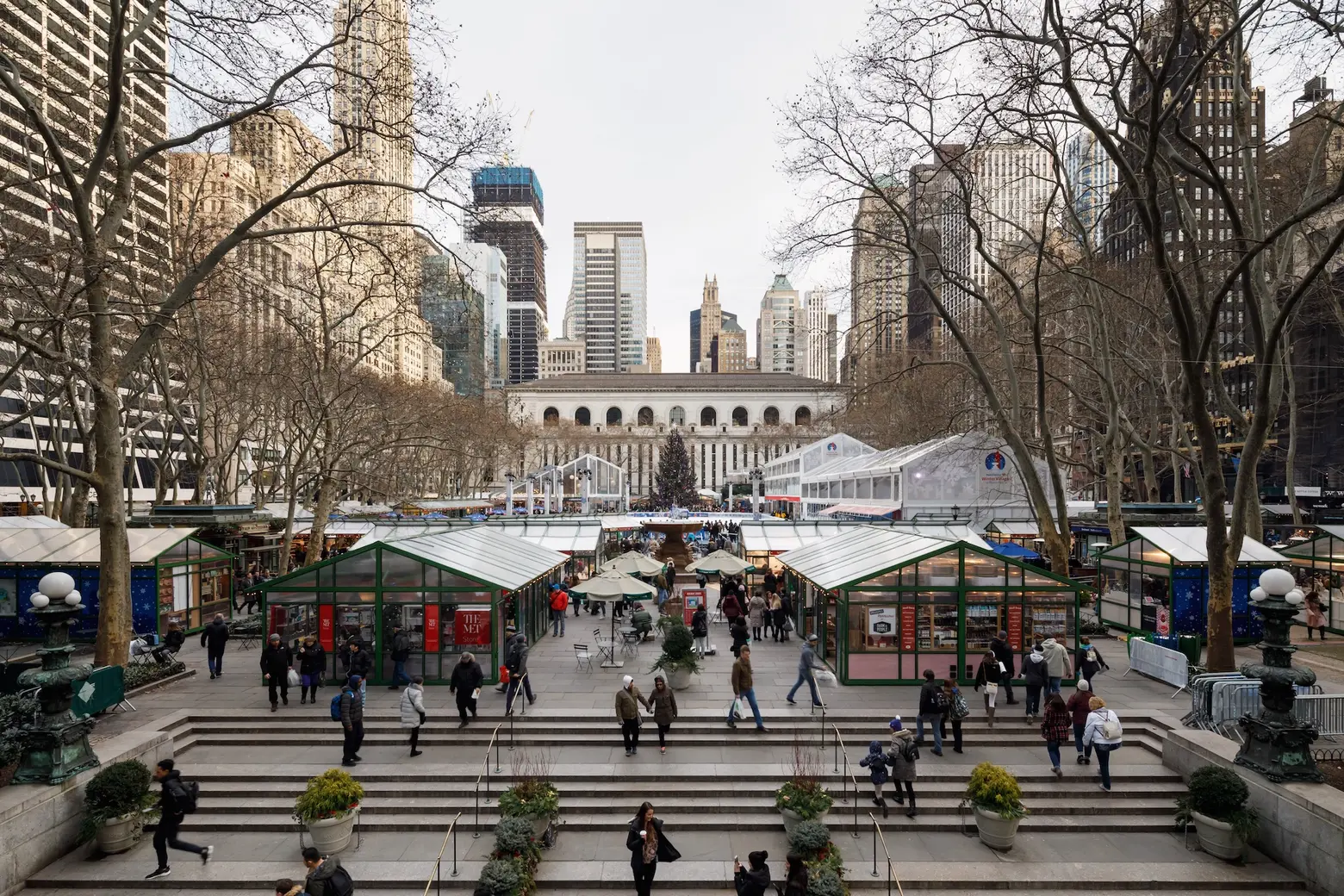The aerial view captures a vibrant open market situated in a large courtyard amidst the towering skyscrapers of New York City, likely in Midtown. This market features a collection of small, glass, greenhouse-like buildings, some of which are multileveled, that host various shops. Steel railings line the short flights of stairs, which have multiple platforms, leading up to the bustling courtyard where many people are seen entering, leaving, and shopping. The seasonal chill is evident from the bare trees positioned on either side of the courtyard, which is dotted with large pots of greenery and contemporary lights. In the center of the image stands a prominent tree, framed by smaller buildings and umbrella-covered tables, all under a clear sky.